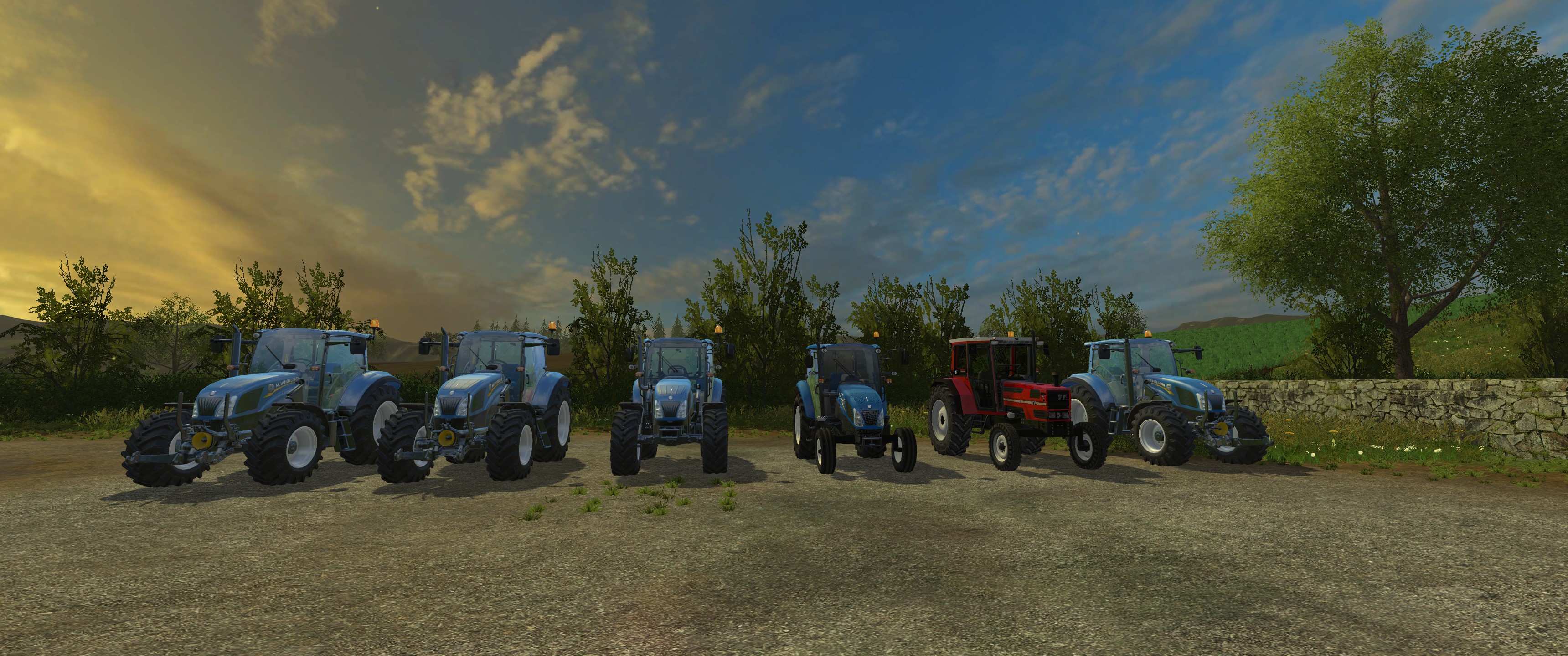The image depicts a vividly detailed animation of a rural scene during either dawn or dusk. The sky is split, with a golden-yellow tint on the left where the sun illuminates the horizon, and a partly cloudy blue sky on the right, featuring light cloud cover. A tree line stretches horizontally across the middle, extending into the upper right corner, with a backdrop of distant mountains. Below, a grassy field transitions into a gravel parking lot, bordered on the right by a stacked grey stone wall. 

In the foreground, six large tractors are neatly arranged in the gravel lot. Five of the tractors are blue, with noticeable variations in size and equipped accessories, featuring black tires with white rims and glass-encased cabs with roofs. The single red tractor, distinct with a white roof over its cab, appears older compared to the others. The composition of the painting highlights the tranquility of a countryside sunset, emphasizing the tractors and their surroundings with meticulous attention to detail.